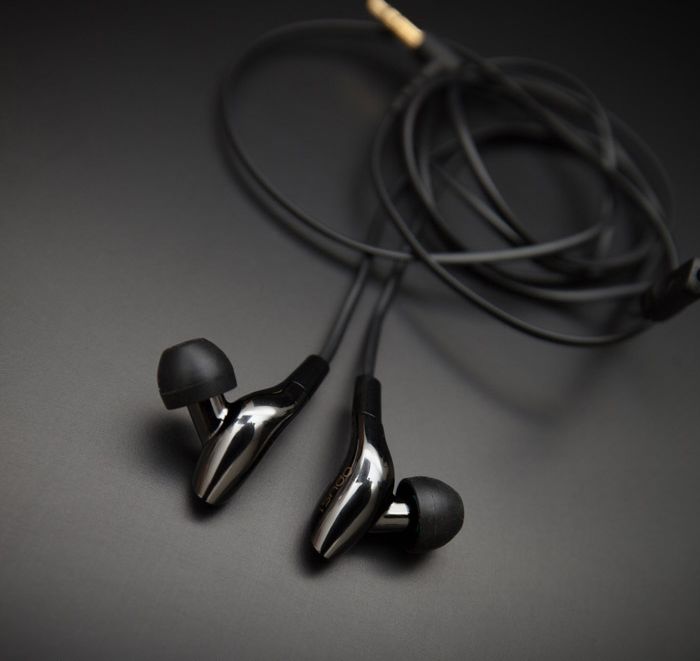The image features a pair of sleek, silver-colored in-ear earbuds with black rubber tips and a short black rubber cable. The earbuds are placed at an angle and offset to the left side of the frame, against a dark gray surface that appears lighter at the bottom due to illumination, likely from a light source. The cord, which is slightly blurred in the background, loops up towards the top and right side of the image, resembling a coiled shape. An L-shaped 3.5mm audio jack with a gold tip is visible behind the earbuds. Additionally, there is an inline volume or mute button discernible on the right side of the frame. The photograph, taken in a macro style, emphasizes the shiny chrome-like aesthetic and banana-shaped stems of the earbuds, creating a detailed and focused close-up shot.